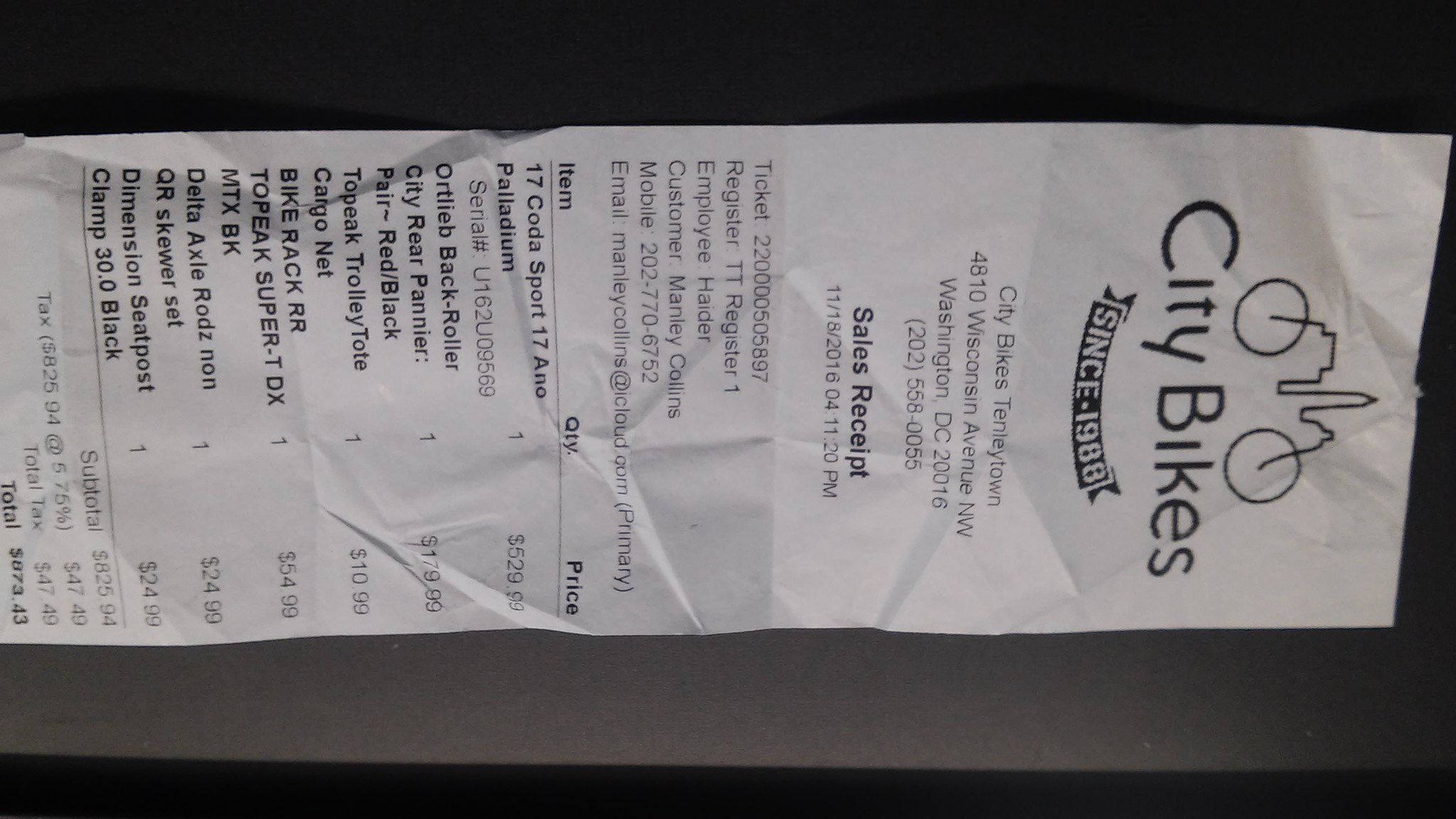This is a photographic image of a long, rectangular receipt that has been scanned in sideways, positioned on a gray background. At the top of the receipt, it says "City Bikes" alongside a logo featuring a bicycle with a cityscape integrated into its frame. Below the logo, a black banner with white text reads "Since 1988." Following this, there's the address and phone number for City Bikes located in Tarrytown, Washington, D.C., along with the label "Sales Receipt" and the date and time of the transaction.

The receipt then lists the items purchased in a vertical arrangement, with each item's name written horizontally in black text. To the right of each item name, the quantity and price are displayed. Notably, one of the items listed is "17 Sports Palladium," contributing to a grand total amount of $673.43, which appears at the bottom of the receipt in black text. Surrounding the receipt image is a background that transitions from black at the top to gray, with the very bottom featuring a strip of black.